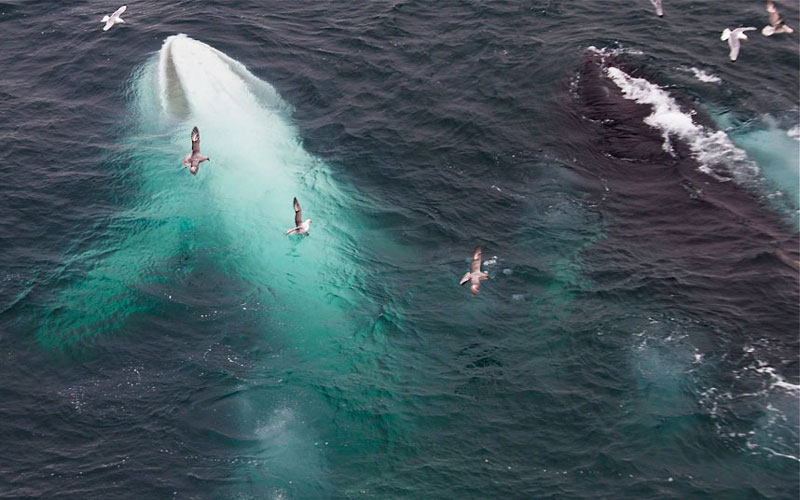This image is an overhead view of the ocean, showcasing a dynamic scene. The deep blue waters are dotted with waves and activity. A variety of seabirds, including seagulls and possibly pelicans, are flying high above, casting their shadows on the water below. Some birds seem to be wheeling around in a somewhat chaotic manner, possibly attracted by the commotion in the water.

In the ocean, two large creatures, likely whales, dominate the scene. On the left side, a white-bodied whale is seen slightly surfacing, revealing parts of its head and torso. Its sleek form creates a distinct ripple in the water, hinting at powerful movement beneath the surface. On the right side, another whale, this one darker in color, is just partially visible. This whale's body remains mostly submerged, but the disturbance in the water indicates its presence as if it might be preparing to surface or breach.

The interaction between the birds and the whales suggests a sense of anticipation in the environment, possibly as if the whales are hunting or the birds are searching for scraps. The overall scene is rich with movement and life, set against the vast, undulating expanse of the ocean.